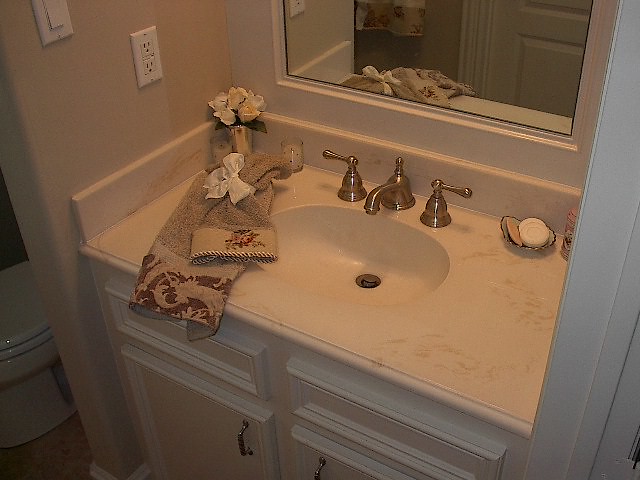A dimly lit, indoor color photograph captures a pristine white marble countertop, either in a kitchen or bathroom, taken from an elevated angle. Central to the image is a stainless steel sink fitted with a polished faucet that features separate hot and cold controls, each with horizontally-oriented handles. To the left on the countertop lies a neatly folded hand towel adorned with a delicate white bow. Just behind the towel in the corner, there is a small silver cup brimming with freshly cut, white roses, flanked by two petite votive candles. On the right side of the sink, nestled against the backsplash, is a soap tray housing three distinct soaps: two circular white ones and an oval tan one. 

In the background on the upper right, a mirror reflects a portion of the countertop, adding depth to the image. To the left, a tan wall is visible, featuring an American electrical socket and a light switch in the upper left corner. Below the countertop, the white cabinet face is visible, complete with metallic handles. Partially in view to the left is a standard toilet, while the edge of a door frame can be seen to the right. The photograph, despite its dim lighting, maintains a high focus on details, emphasizing the serene, organized, and elegant arrangement of the space.